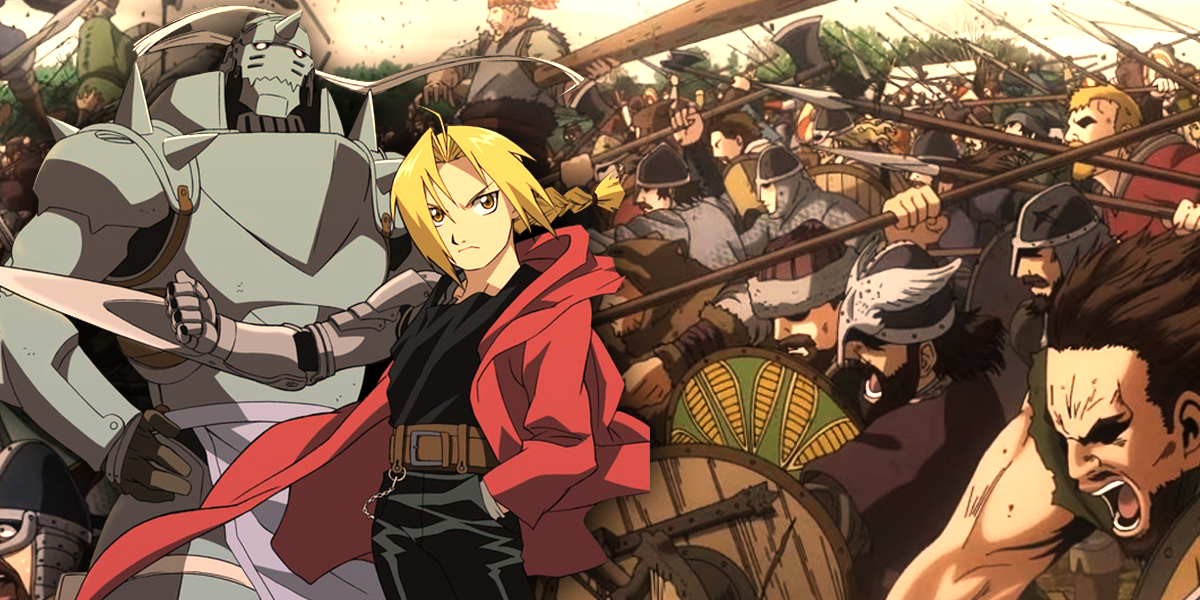This detailed and vibrant image captures a dramatic battle scene from the anime Fullmetal Alchemist. At the forefront on the left side, stands the main character, Edward Elric. Edward is a young man with shoulder-length blonde hair and an intense, menacing expression directed at the viewer. He is wearing a red trench coat that flows like a cape, a loose black shirt, and shiny black pants. A large brown belt with a chain hanging from it cinches his outfit. His left hand is tucked into his pocket while his right arm is a futuristic metal prosthetic, ending in a blade protruding defiantly from his wrist.

Standing imposingly behind Edward is his brother Alphonse Elric, a towering figure encased entirely in a gigantic suit of gray armor. Alphonse's armor design is intricate, complete with a ribbon streaming from his head and a purple loincloth, making him resemble a robot or a medieval knight.

On the right side of the image, the background is alive with an intense and chaotic battle scene. A large throng of medieval-style warriors, clad in plate armor and capped helmets, charge forward with open mouths in mid-battle cries. They wield long spears, axes, and shields decorated with green and yellow designs or plain wood. The scene also includes a colossal figure in the center top of the image, hoisting a massive wooden beam. There are hints of greenery and sunlight towards the top, indicating an outdoor setting amidst the clash of these fierce combatants.